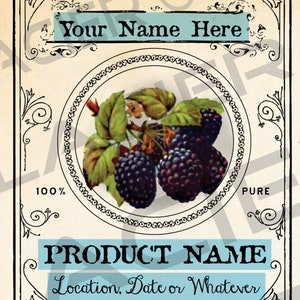This image features a meticulously detailed illustration of a vintage-style label on yellowed, aged paper, adorned with elaborate line work and ornate scroll designs. Central to the label is a circular emblem that showcases a realistic depiction of blackberries surrounded by leaves. Flanking the circle on either side, the words "100% pure" are prominently displayed. At the top, a light blue banner with the customizable text "Your Name Here" stands out in black letters. Below the circle, "Product Name" is written in bold, capital letters on the same blue banner. Further down in a script font, there is a section for adding the location, date, or other details, maintaining the continuity of the blue banner theme. A watermark runs across the entire image, adding to the authenticity of the vintage design. The label is bordered with intricate patterns that frame the entire layout elegantly.